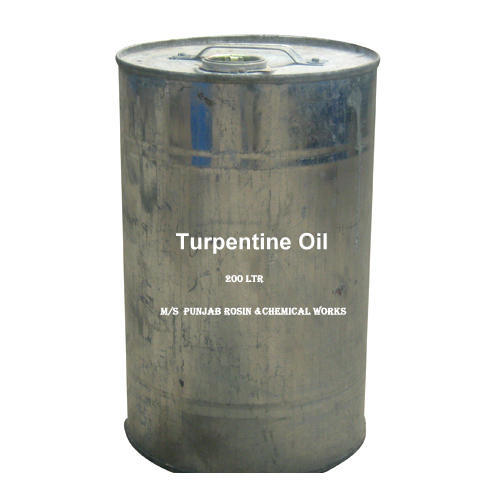The image depicts a large, dirty, dull gray canister with a distinct, interconnected handle and a circled spout on top. The can features a white label in the center that reads "Turpentine Oil" with the words capitalized at the start. Beneath this title, in smaller text, it specifies "200 LTR," indicating the capacity of the can in liters. Further down, the label reads in all capital letters, "M/S Punjab Rosin and Chemical Works." The can itself is largely silver, marred with streaks of dark gray, and there is a noticeable blue strip near its top. The scene suggests an industrial or outdoor setting, likely a factory, indicative by the can's soiled appearance and utilitarian design.